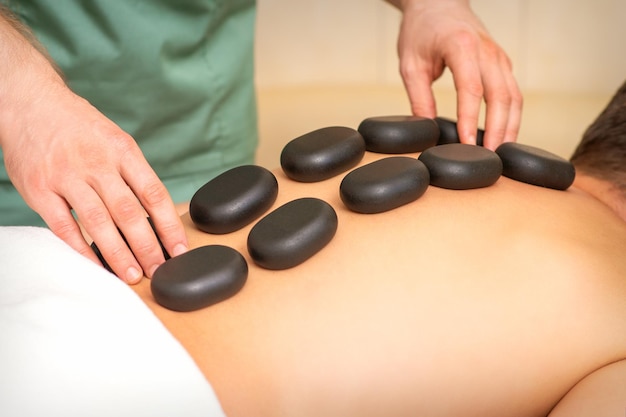The image depicts a man receiving stone therapy. He is lying on his stomach, his head positioned towards the upper right corner of the image and his waist toward the lower left. A towel is draped around his lower body. His shirtless back arches gently, and arranged along his spine are ten flat, oval-shaped rocks, divided into two parallel rows stretching from the neck down to the waist. Standing beside him, a therapist wearing a green uniform, resembling surgical attire, carefully positions the stones on the man's back. The therapist, whose face is out of frame, places both hands on the stones, possibly to adjust them or apply treatment. The background is a simple, blurred gradient from white to tan, providing no additional context to the setting.